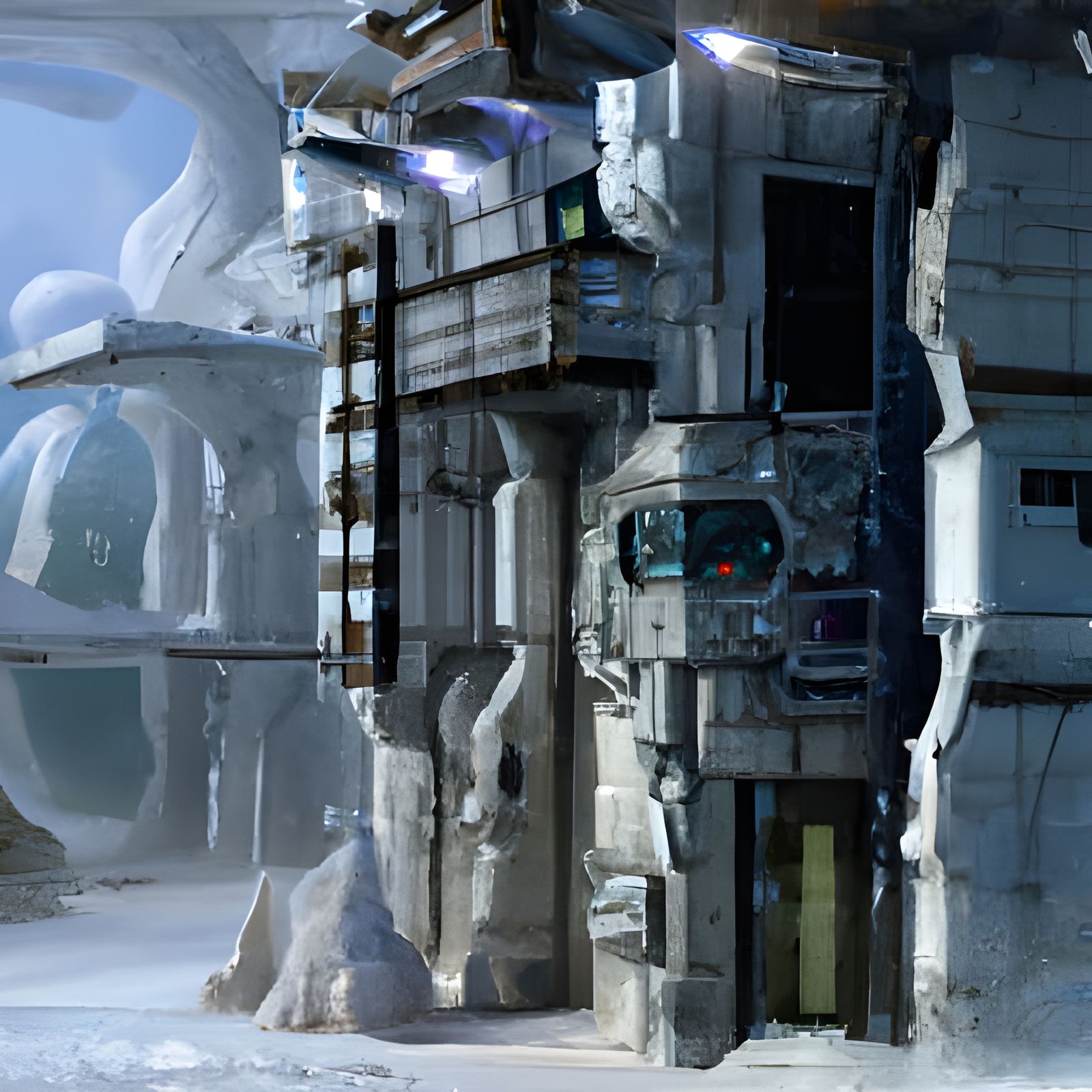The image depicts a futuristic, wintry scene, possibly from a science fiction movie, an AI-generated scenario, or a high-end video game. The foreground features a large, cement-like structure with numerous jutting elements and a rounded dome overhang. A striking feature is a bright green panel embedded in what appears to be a doorway on the lower right. A glass-like door with a red and blue center dot is also visible, hinting at some sort of control panel or observation post. Adjacent to it are narrow windows and a ladder-like structure on the center left, enhancing the industrial look. The ground is littered with chunks of ice and snow, emphasizing the frigid climate. The background showcases a light, hazy blue sky and additional curved, high-tech buildings, lending an abandoned yet advanced look to the scene. The environment is entirely devoid of people, adding to its desolate and cold atmosphere.